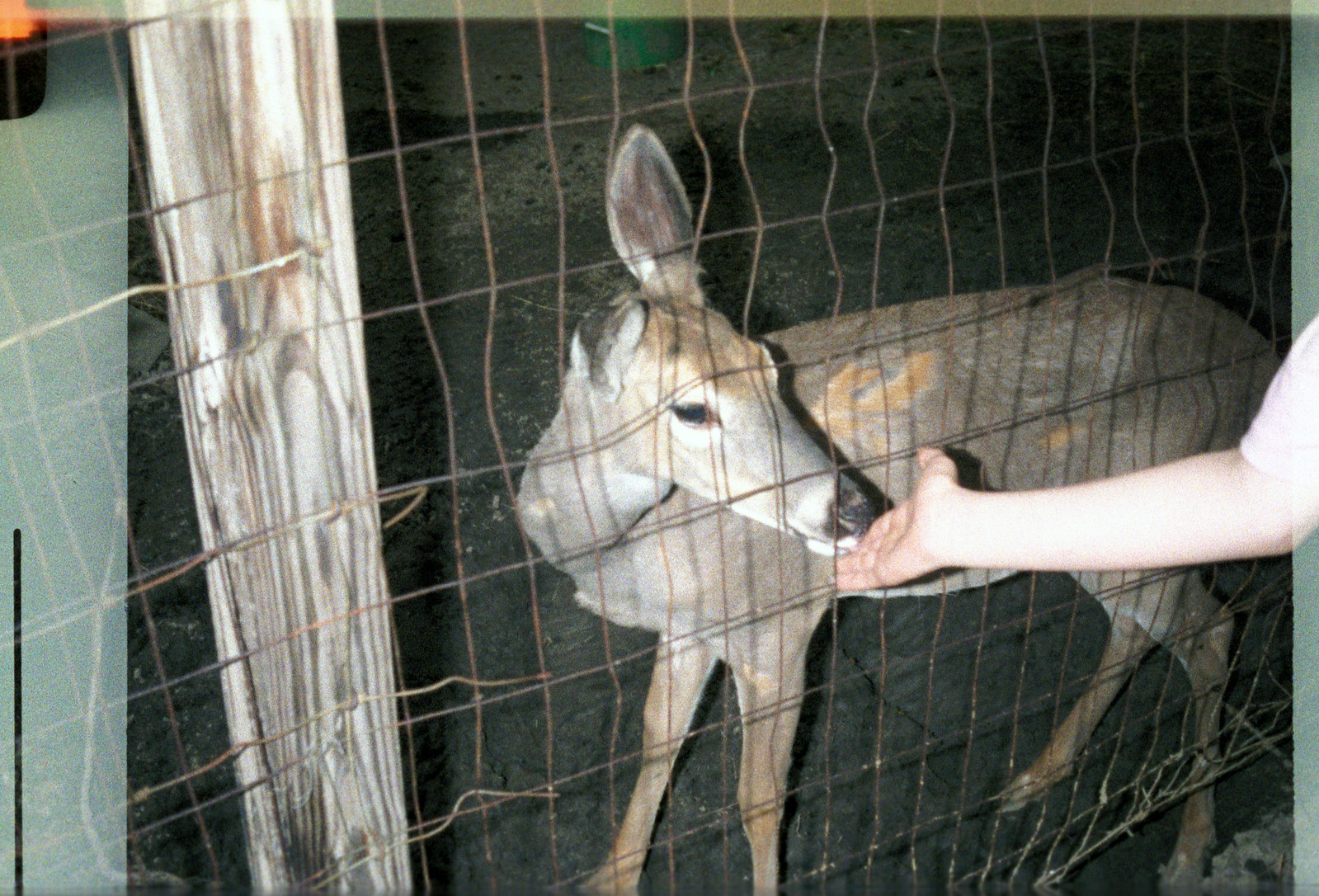In this image, a person extends their hand through a rusted, rectangular wire mesh fence to feed a brown deer with lighter orange patches on its back and thigh. The deer's body faces left, but its head is turned slightly right towards the hand, touching it with its nose. The fence is attached to a wooden post on the left side of the picture. You can see the person's arm coming from the middle right side, with the forearm and palm visible as they offer food to the deer. The image includes a thin gray border on the right side, sections of light blue on the far left, and an orange and black object at the very top. Notably, it appears the deer may be missing one ear, as only one ear is visible on the right side of its head. The setting resembles a farm, indicated by the visible dirt on the ground.